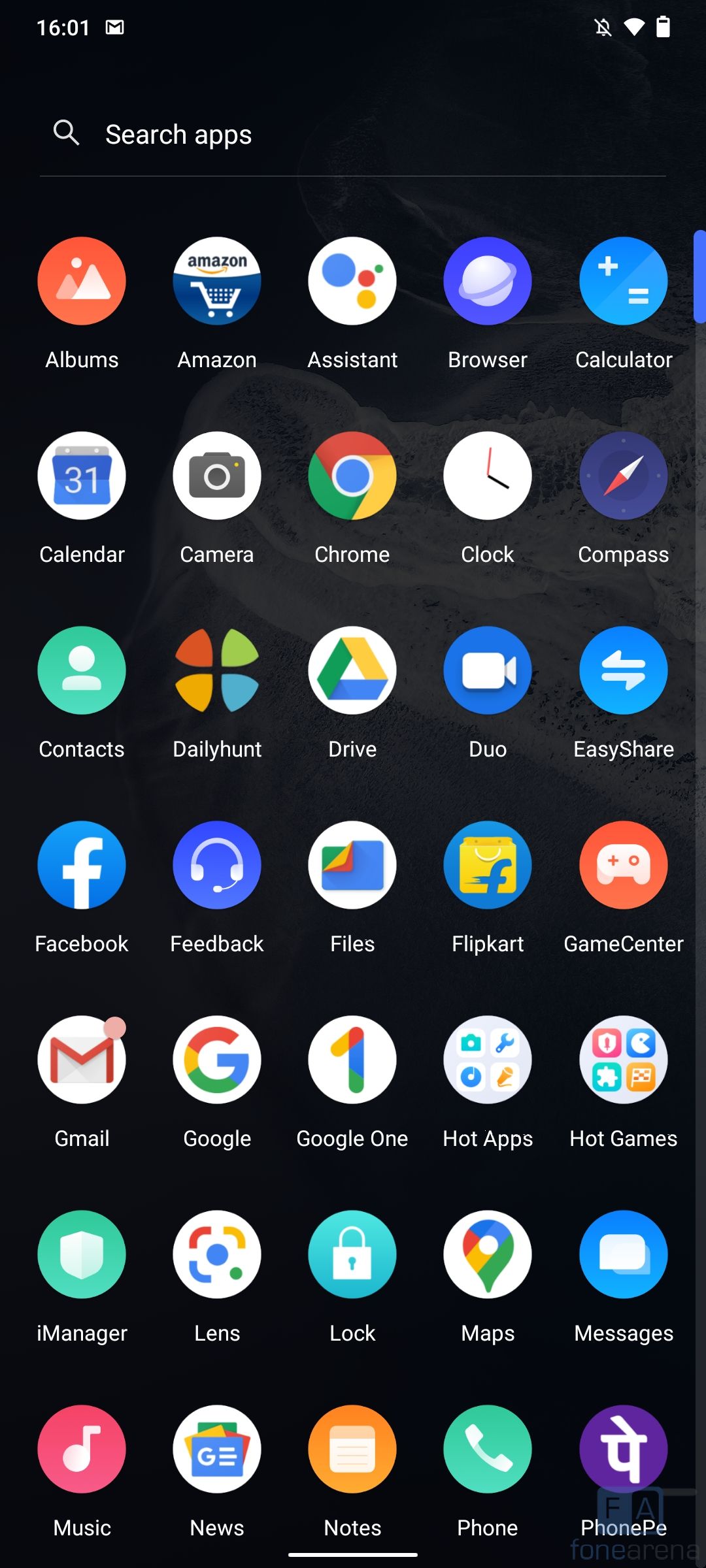This image is a screenshot of the apps page on a mobile phone, taken at 16:01 with the battery at approximately 75% charge. The phone is connected to Wi-Fi. The background is black, and at the top of the screen, there is a search box labeled "Search apps." The page is filled with a diverse array of colorful app icons, including Albums, Amazon, Assistant, Camera, Chrome, Clock, Calendar, Compass (listed twice), Contacts, Drive, Duo, Facebook, Files, Notes, Phone, Lock, Lens, and Gmail, among others. This extensive collection of apps demonstrates the necessity of the search function to navigate through them efficiently.